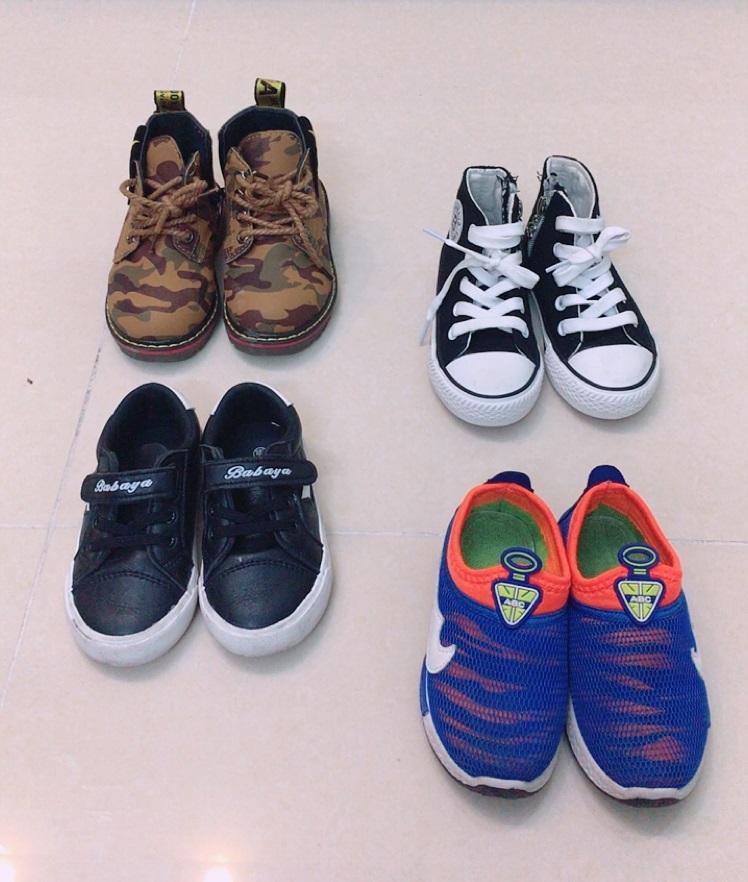This photograph showcases four distinct pairs of toddler shoes neatly arranged in a quadrant on a pristine white floor, accentuating the vibrant colors and designs of each pair. The top left quadrant features camouflage-inspired boots, reminiscent of Doc Martens, with khaki, green, and brown prints and thick rope-like laces. Directly to the right, in the top right quadrant, are a pair of high-top Converse-style sneakers, adorned with white laces and zippers on the sides for easy access, exhibiting a classic black and white color scheme. In the bottom left quadrant, there is a pair of black low-top sneakers with Velcro closures, branded "Babaya" on the straps, and a white sole base. Completing the set, the bottom right quadrant displays blue slip-on sneakers highlighted with orange accents around the opening, and marked with the logo "ABC" inside a yellow triangle.